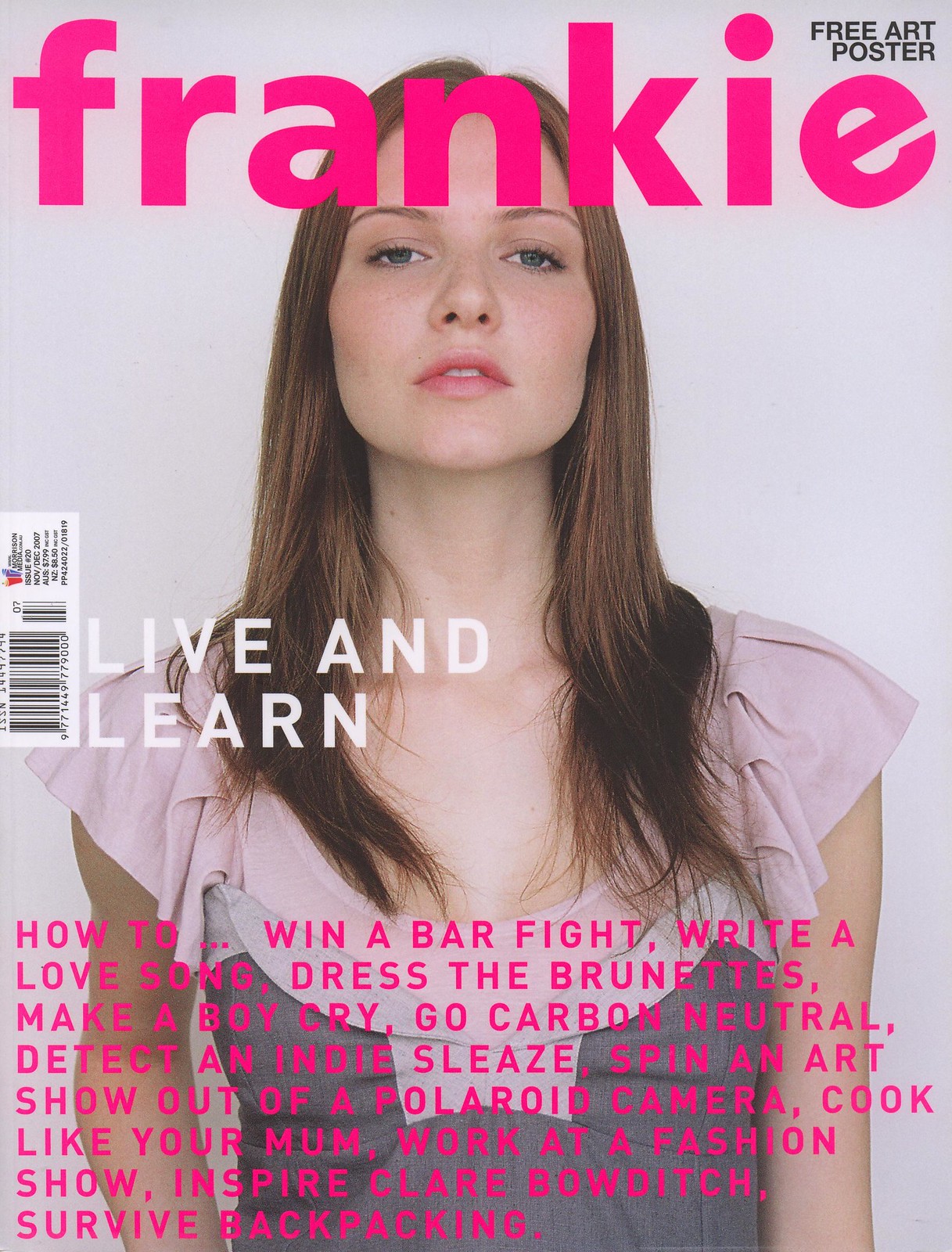The magazine cover features a prominently centered image of a very thin, pale-skinned woman with long, straight brown hair that falls slightly past her shoulders. Her light grayish-blue eyes stare directly into the camera, and she has a slightly raised chin, giving her an assured and composed look. She is wearing a scoop-neck top with no sleeves; the top part of the shirt is made of a pink and white poofy fabric, while the section from her chest down is gray, suggesting a two-tone design.

The background of the cover is a light gray, providing a neutral backdrop that accentuates the subject's features. The title of the magazine, "Frankie," is displayed prominently at the top in large, hot pink lowercase letters. In the top right corner, in small black text, the phrase "free art poster" can be seen. Scattered across the cover, various other headlines draw the reader's attention, including "live and learn," and a series of phrases in hot pink text at the bottom that read: "how to win a bar fight, write a love song, dress the brunettes, make a boy cry, go carbon-neutral, detect an indie sleaze, spin an art show out of a Polaroid camera, cook like your mom, work at a fashion show, inspire Claire Bowditch and survive backpacking."

Overall, the cover blends stylish design with intriguing, lifestyle-oriented headlines, perfectly capturing the essence of a contemporary fashion and lifestyle magazine.